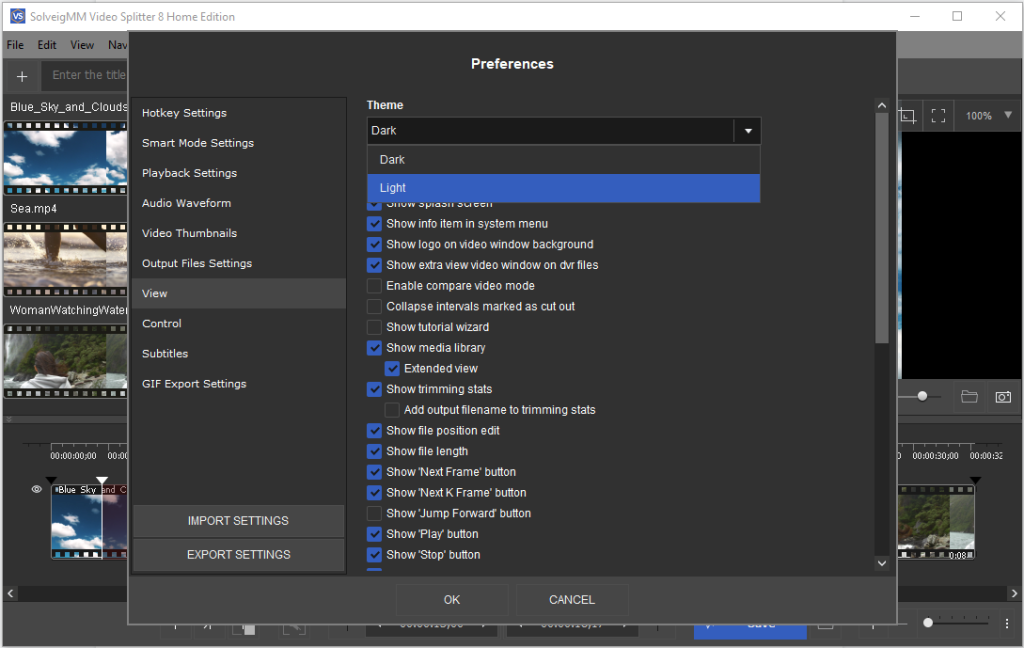In this image, we see the interface of a video editing software called "Solvay MM Video Splitter 8 Home Edition," prominently displayed at the top-left corner. The software is identified by a blue icon with the letters "VS" written in white. On the left of the screen, there is a preview window showing video footage of the sea and a woman watching the water. The right side of the screen showcases the Preferences settings panel.

The Preferences panel features a sidebar menu in white text, listing various settings: Hotkey Settings, Smart Mode Settings, Playback Settings, Audio Waveform, Video Thumbnails, Output File Settings, View, Control, Subtitle, GIF, and Export Settings. At the bottom of this sidebar, there are two buttons labeled "Import Setting" and "Export Setting."

The currently selected menu is "View," which is highlighted. In the View settings, there is a dropdown menu for selecting the theme. Although the menu reads "dark," indicating a potential option, the selected theme is "light," distinguished by its blue highlight. 

Below the theme selection, various other view preferences are displayed with toggle options:
- Show Information (ON)
- Info Item in System Menu (ON)
- Show Logo on Video (ON)
- Window Background (ON)
- Show Extra View (ON)
- DVR Files (ON)
- Enable Compare Video Mode (OFF)
- Collapse Interval Markers (CUT OUT)
- Show Tutorial Wizard (OFF)
- Show Media Library (ON)
- Show Trimming State (ON)
- Show Files Positioning (ON)
- Show File Length (ON)
- Show Next Frame Button (ON)
- Show Next Key Frame Button (ON)
- Show Jump Forward Button (OFF)
- Show Play Button (ON)
- Show Stop Button (ON)

The overall layout captures the sophisticated and detailed user interface of the video editing software, highlighting its user-friendly options and extensive customization capabilities.